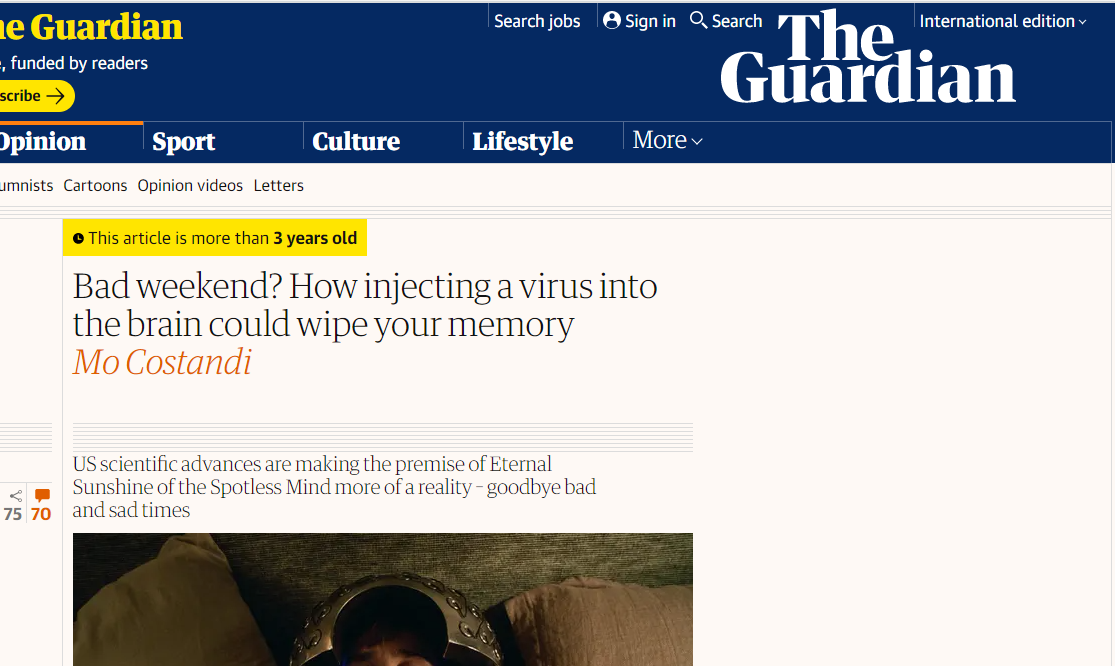A detailed and cleaned-up caption for the image you described could be:

"The image is a cropped screenshot of a news or magazine website, identified as 'The Guardian.' In the top left corner, partially cut off, is 'The Guardian,' with only the 'E' and 'Guardian' visible in yellow. A truncated subscription button is visible, although it is partially cropped out. On the right side, 'The Guardian' is displayed in white. Four links are aligned at the very top left: 'Search jobs,' 'Sign in,' 'Search,' and 'International edition.' A blue bar spans the top, just below these links, containing a top menu with buttons labeled 'Opinion,' 'Sport,' 'Culture,' 'Lifestyle,' and 'More.' Below this menu, an article is featured with a prominent yellow tag indicating 'This article is more than three years old.'"